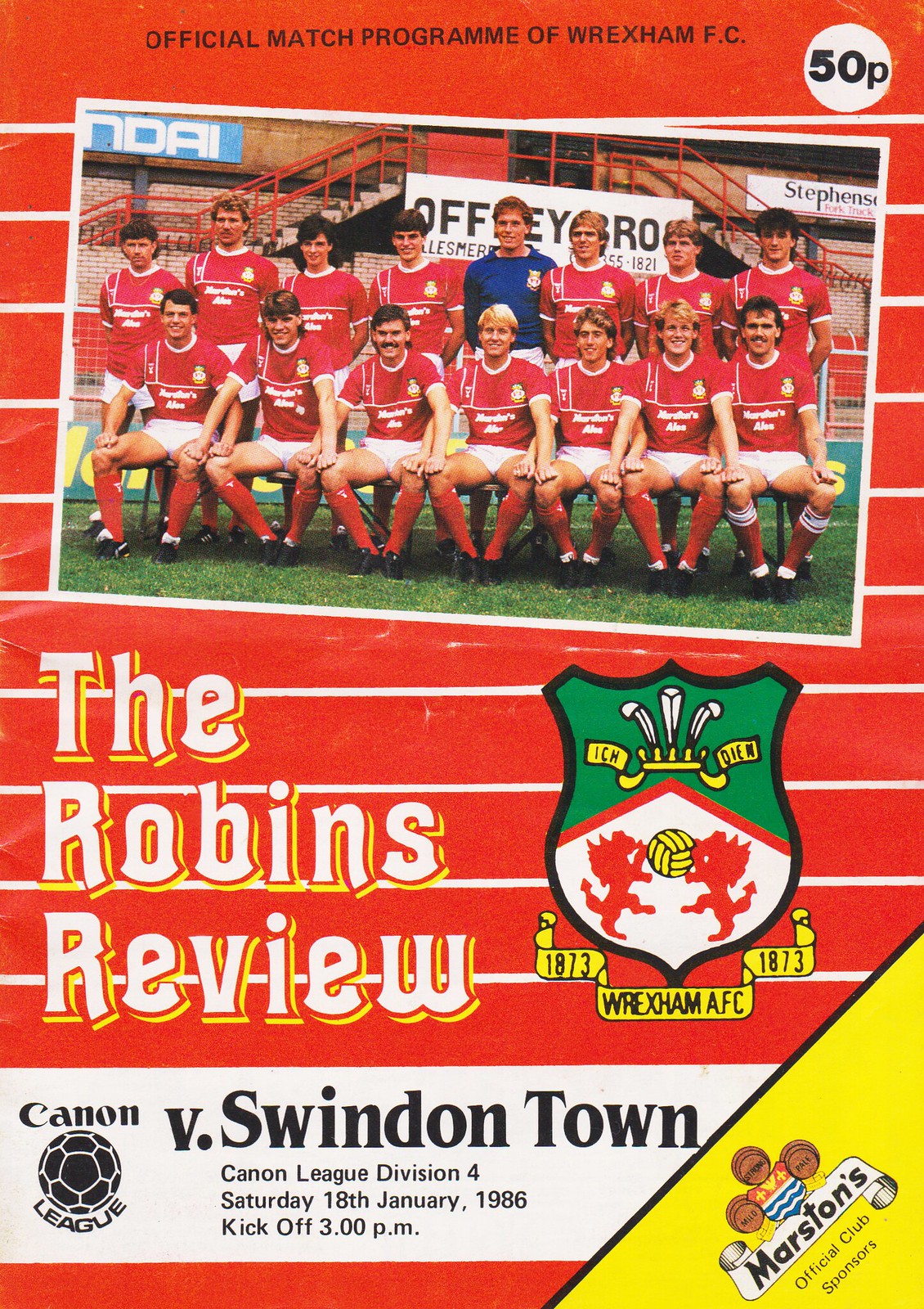The cover of the magazine is predominantly red with horizontal white stripes. At the top, black text reads, "Official Match Program of Wrexham FC," with a white circle nearby indicating the price of 50p. Below, a large historical photograph of a soccer team from circa 1873 features players wearing red shirts with white shorts and red socks. The team members, posed for the photograph on a grassy field, have badges on their chests and a player stands prominently in the center in a blue shirt. In the background of the photograph, the words "NDAI" in white on a blue background and "Stevenson" in black on a white background are visible. Beneath the image, the title "The Robins Review" is displayed alongside a badge featuring green and white colors with two lions fighting over a blue soccer ball. Details about the match follow, stating, "Canon League V. Swindon Town, Canon League Division IV, Saturday, 18th January 1986, kickoff at 3 PM." In the bottom right corner, a yellow triangle highlights "Marston's Official Sponsors" with the Marston's logo of three coin-shaped circles, a shield, and the name "Marston's" on a ribbon.